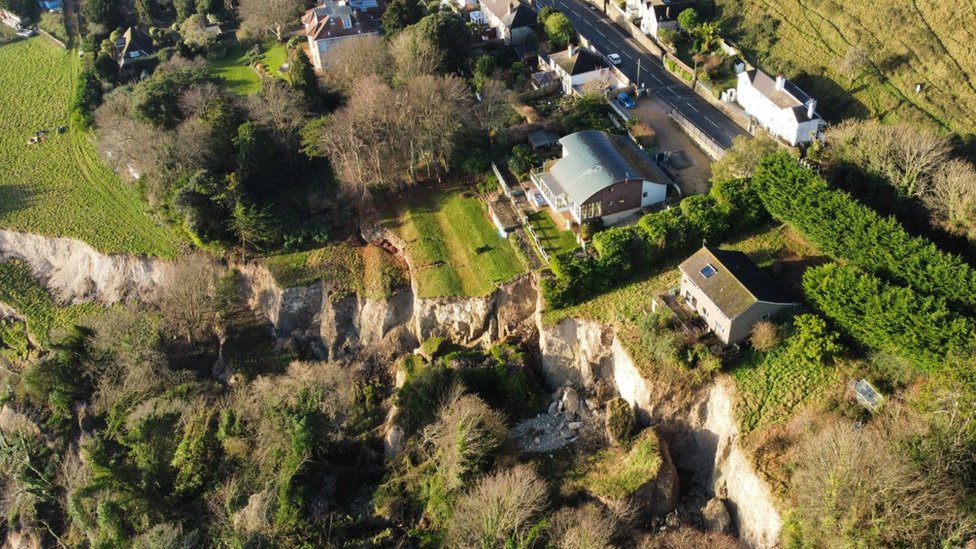This is a daytime aerial color photograph of a farm nestled on a hillside and extending into a valley, prominently divided by a cliff running from the left side of the image to the center, where it makes a sharp turn down to the foreground. The central focus is a large barn with a metal round roof, set among numerous outbuildings connected by a road and surrounded by lush vegetation. The land features an array of short green plants as well as taller trees, some of which are leafless, hinting at a spring or fall season. 

In the upper area of the image, a long white building, possibly residential, sits across the road from the barn. Behind the barn, terraces shape the landscape, and a smaller white structure with a skylight is closer to the viewer. On the right side, a house with a brown roof and beige front is partially enclosed by hedgerows, which wrap around to leave a small backyard area. Nearby, a large green tree and a smaller browned tree are visible among multiple bushes.

The lower left corner exhibits a dense collection of trees and brush, with some browned vegetation indicating seasonal change. Adjacent to this area, several homes on the hillside feature pitched brown roofs and are closely bordered by trees that have shed their leaves. Dotted among the buildings and extending towards the foreground, other houses and outbuildings are interspersed with clearings and further vegetation. The road on the upper right runs diagonally, lined with white and brown-roofed houses and a few visible cars, blending into the expansive, vegetated landscape.